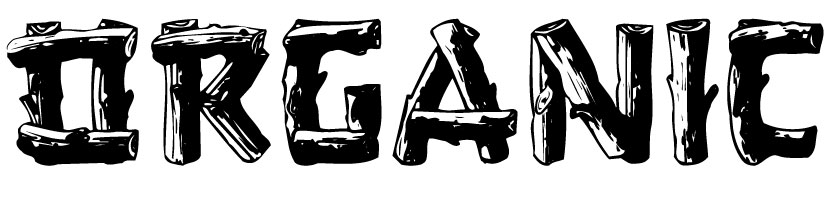This is a black-and-white, artistic image featuring the word "ORGANIC" spelled out in all capital letters. The composition is set against a plain white background. Each letter is creatively constructed from cartoon-like logs, lending a whimsical and hand-drawn quality to the design. Specifically, the "O" is formed by four logs arranged in a rectangular manner, while the "R" includes a vertical log on the left, a curved log on the top right, and a diagonal log forming the leg. The "G" consists of three logs with the top part of the right log cut off. The "A" appears as a triangle of three logs, slightly elevated so the legs extend outward. The "N" is constructed with logs on either side and one log slanting diagonally in the middle. The "I" is a singular log standing upright, and the "C" uses three logs arranged to form its curved shape. Overall, the illustration emphasizes the natural theme through its log-based letter forms, and although it's not photorealistic, the cartoonish style gives it a distinctive and engaging appearance.